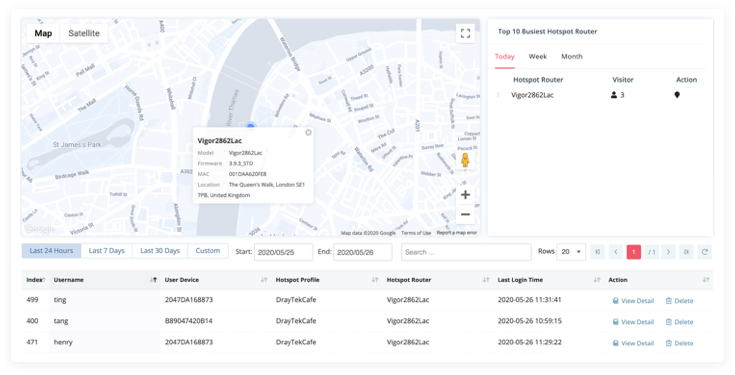This image depicts a hotspot heat map on a white background, providing detailed information about a specific router and its usage statistics. 

In the upper left corner, a map occupies approximately the top third of the image. The map highlights the location "Vigor 2862 LAC," along with details including the model type, firmware version, MAC address, and the specified location, which is in London, United Kingdom. More precisely, the map indicates an area near Queen's Walk, between St. James Park and about a mile or two east of it. The bottom part of this section displays the text "79P United Kingdom" and "London" for further location specificity.

The map view is in dark mode, indicating that the selected view is "Map," as opposed to "Satellite," which is an available option situated to the upper left. Adjacent to this, on the upper right, the text "Top 10 Busiest Hotspot Routers" is visible, followed by options for viewing data from "Today," "Week," and "Month," with "Today" highlighted in red and underlined.

Beneath these headings, the specific hotspot router is identified again as "Vigor 2862 LAC." This section also indicates that there are three visitors currently connected to it, marked next to the label "Visitor 3," accompanied by an action icon resembling a location pin.

Further below, there are various search parameters available for more refined data analysis. These include "Last 24 Hours," "Last 7 Days," "Last 30 Days," "Custom," along with options to select a start and end date, and a search button. The "Last 24 Hours" option is currently highlighted. 

The final part of the image lists three usernames, likely representing the visitors connected to the hotspot router at the Dre Tech Cafe.